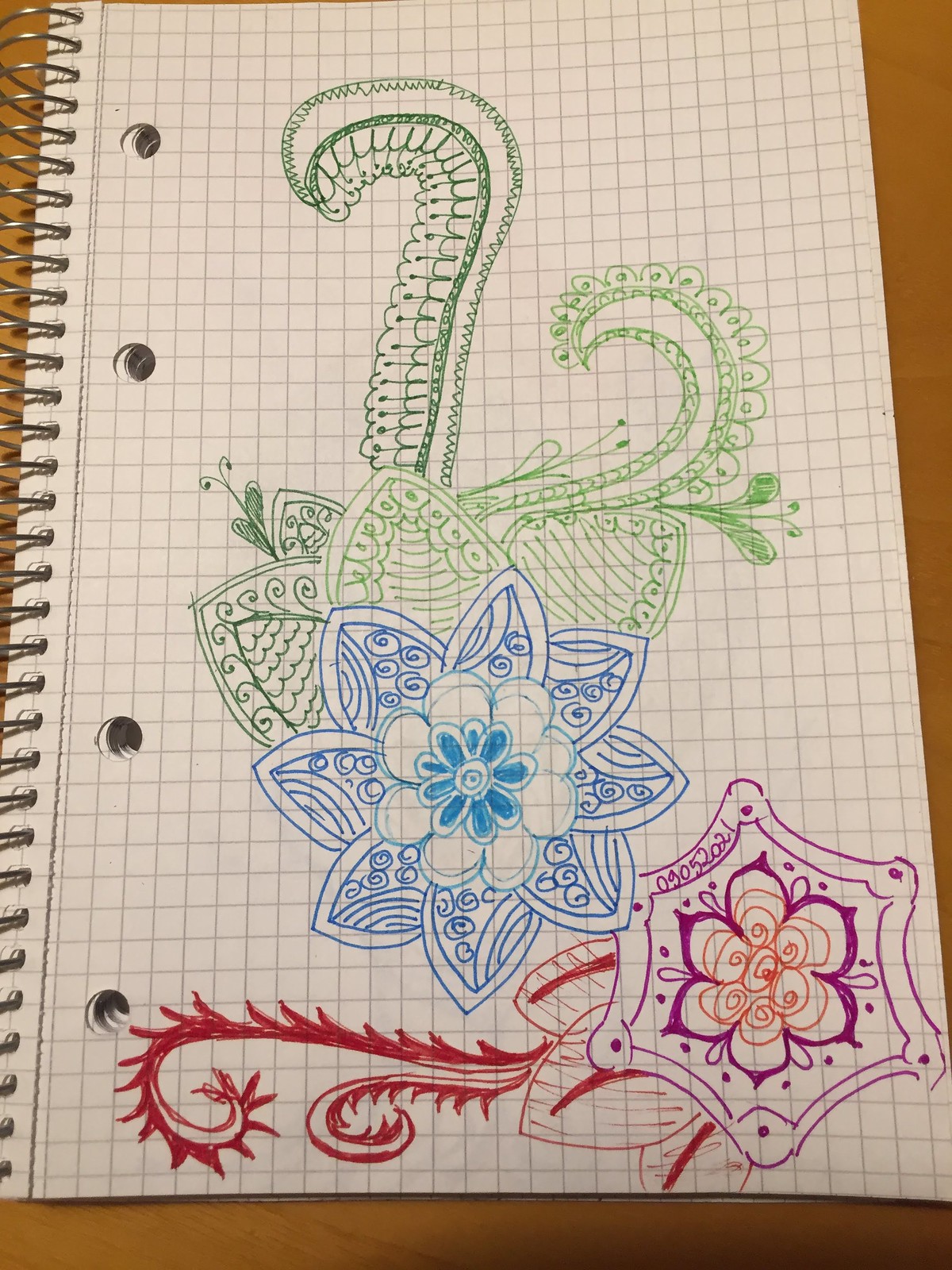The image is a drawing rendered on a square type of notebook paper, distinguished by the visible metal wire binding on the left-hand side, which is captured at a slight angle. The artwork prominently features two unique elements that appear to blend the aesthetics of flowers and dragon tails.

At the bottom of the drawing, there is a horizontally positioned element. This appears to be a hybrid flower-dragon tail, with the flower's face oriented towards the lower right corner. The tail extends outward, curling towards the bottom left side of the page.

Above this element, centrally positioned, is a second flower-dragon tail hybrid. This upper element features a vibrant blue flower. From the center of this flower, the tail extends vertically upwards, reaching towards the top of the image. The contrast of colors and the flowing nature of the tails create a dynamic and visually engaging composition.